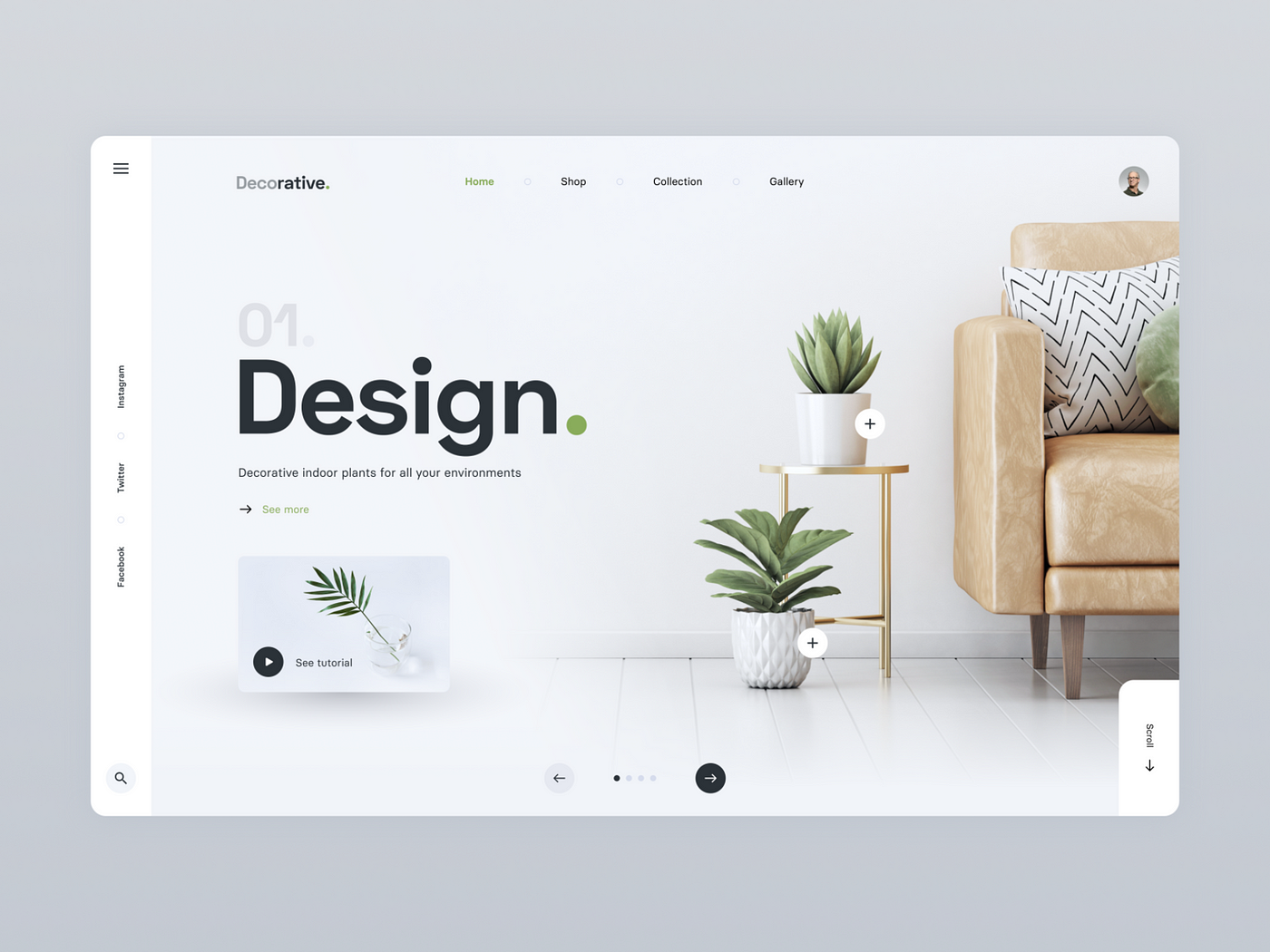This image appears to be a catalog or homepage from a design company's website. The layout features a clean, modern aesthetic with a predominantly white background, gray accents, and minimalistic text. At the very top, navigation options include "decorative," "home," "shop," "collection," and "gallery." The brand name "decorative" is prominently displayed in the top left corner.

Centrally, the page displays the number "01" in large black font against a white section, followed by the word "design" in bold black, and a tagline in smaller black text: "decorative indoor plants for all your environments." Below this text section, within a white box, there's an insert featuring a glass vase filled with water and a single leaf, accompanied by the phrase "see tutorial."

To the right of this insert, a gold metal side table is adorned with a white vase containing an aloe-like succulent, while another white vase with a green plant sits directly on the floor. Adjacent is a tan leather sofa, with just the edge visible, complemented by two pillows: one with black and white zigzag stripes, and a green round pillow. The walls and floors are predominantly white, enhancing the minimalist and contemporary feel. Complete with clickable plus signs for adding items to a cart, this page effectively marries functional e-commerce elements with sophisticated design.